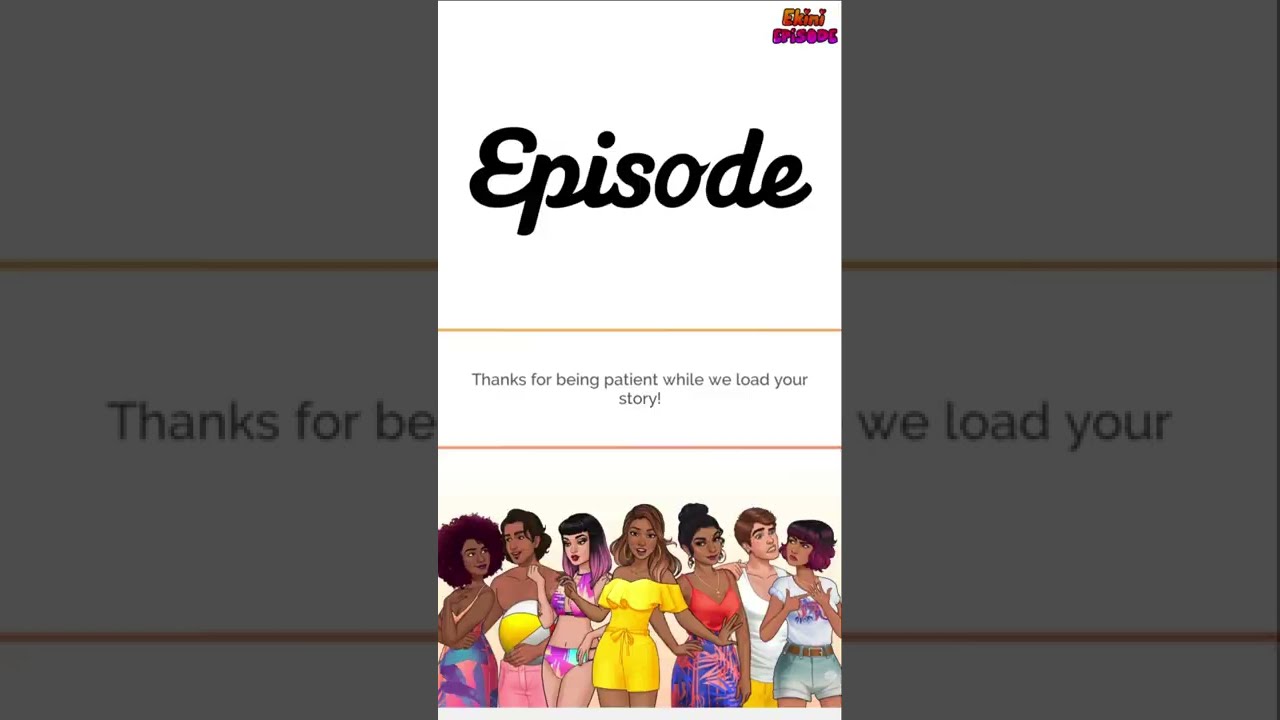The image is a screen capture from an app, specifically titled "IKINI EPISODE" at the very top right corner in cartoon letters. Directly beneath the title, in a decorative black cursive font, it says "EPISODE" on a white background. Across the center of the screen, enclosed between two thin lines—a light pink one and a tan one—is the message: "Thanks for being patient while we load your story."

Below this message, a variety of diverse, cartoon-style characters are illustrated. These characters appear to be young men and women of different ethnicities, dressed in a mix of beachwear and stylish outfits, including bikinis, swimsuits, shorts, tank tops, and sarongs. Notable among them are a girl with purple hair, a lady with an afro wearing a pink and purple skirt, and a man holding a beach ball while dressed in pink shorts. The characters are engaging in interactions such as whispering, talking, and flirting with each other, suggesting a lighthearted, social, and possibly romantic theme akin to a "90210" scenario. The overall layout includes a bordered section created from the grayed-out area around the central message, enhancing the visual structure of the image.